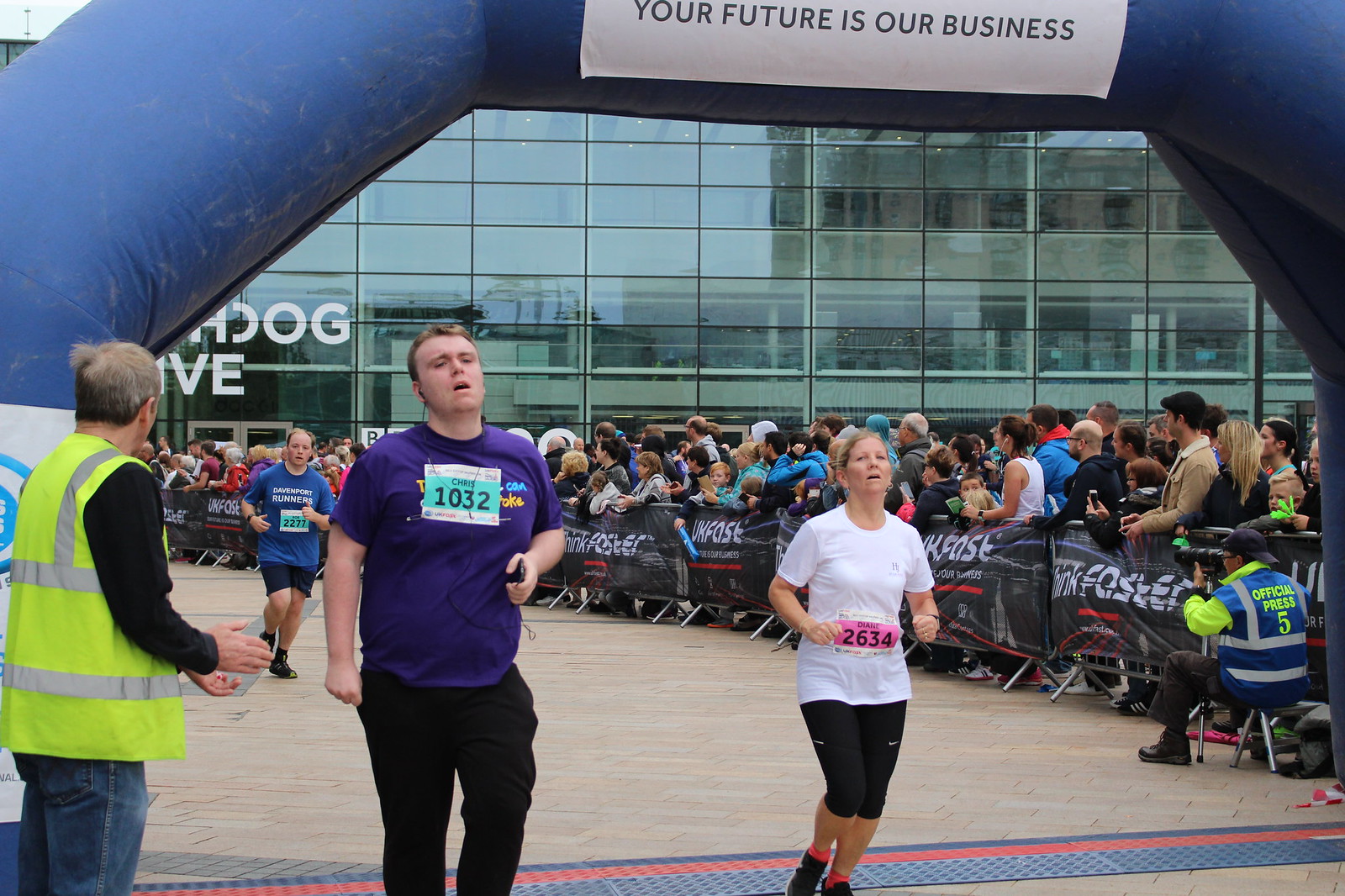In this photograph capturing the exciting conclusion of a road race, two central runners—Chris and Diane—are finishing strong under an inflatable blue finish arch that prominently displays the message "Your future is our business" in bold black text. Chris, positioned on the left, sports a short-sleeved purple t-shirt and dark pants, with his race bib number 1032 easily visible alongside his name. Diane, to his right, wears a white short-sleeve top and black pants, identified by her bib number 2634. Just behind them, another male runner in a blue shirt strives to reach the finish line. The background features stands packed with vibrant spectators, cheering behind barriers, adding to the lively atmosphere. A man in a high-visibility yellow vest stands to the left, ensuring the event runs smoothly. Flanking the runners and the energized crowd is a large building, completing the engaging scene of this triumphant race finish.